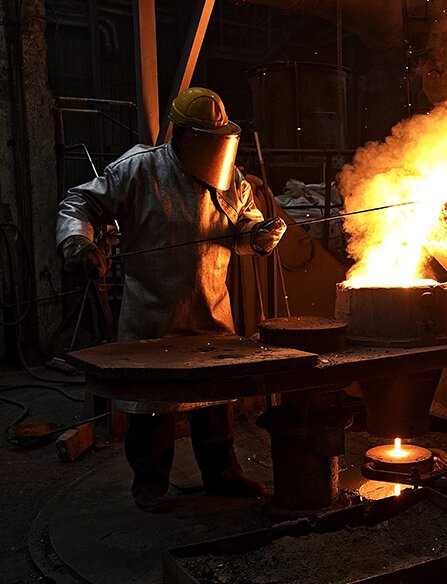In the dim, industrial backdrop of a dark room filled with pipes and containers, a figure clad in a heavy, silver fireproof suit and a large welding mask stands at a sturdy worktable. Bathed in the glowing light from a large flame emerging from a stone pot, the figure holds a thin, two-foot long metal rod over the searing heat. With gloved hands steady, they tend to the liquid metal that drips from the pot onto a plate below, suggesting a meticulous process of welding or metalwork, potentially even sword-making. The intense brightness of the flames contrasts with the surrounding darkness, highlighting the craftsmanship and the protective gear that shields the person from the fiery sparks and molten materials.